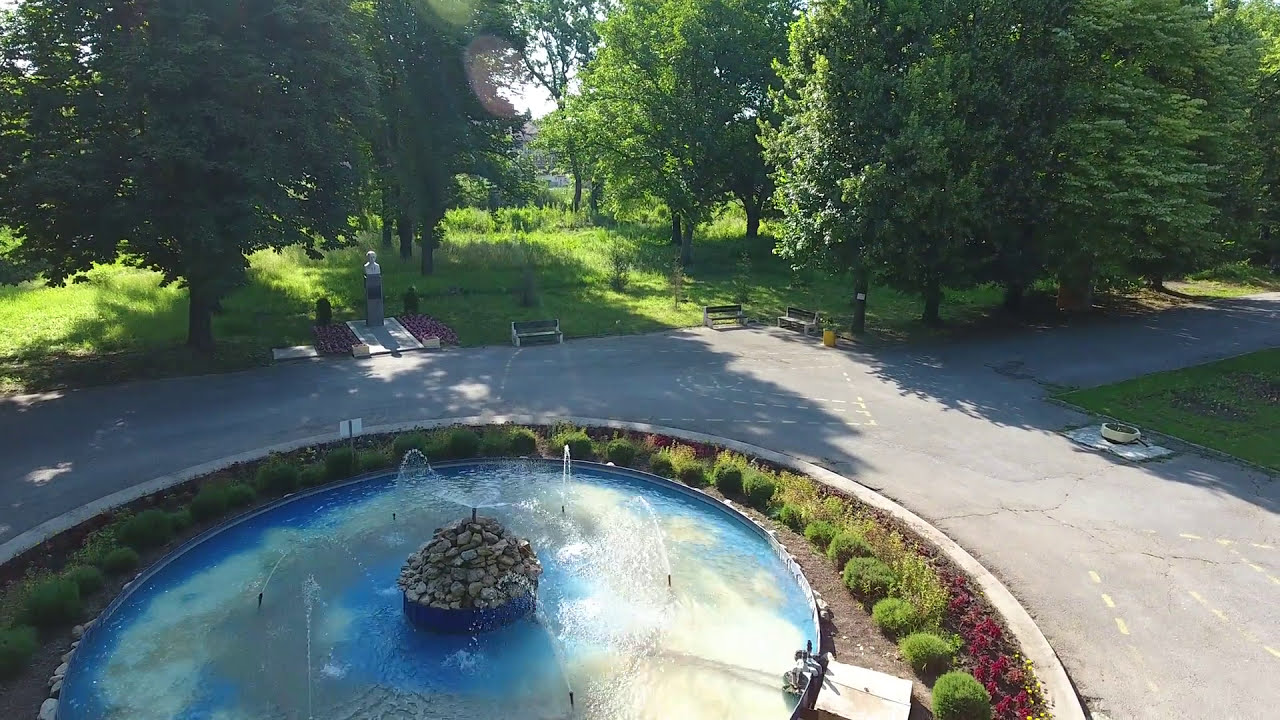The photograph captures a picturesque scene in a park dominated by a circular fountain at the lower left and center of the image. This fountain features a central stack of rocks with a water sprayer that reaches about three feet high, surrounded by six smaller sprayers creating a symmetrical water display. Encircling the fountain is a meticulously maintained arrangement of greenery and red flowers, enclosed by a cement border. This border integrates seamlessly with a gray path, which branches off to the right and left, inviting exploration. The park's landscape is lush with grassy areas and tall pine trees, creating a serene backdrop. Adding to the charm, there are benches positioned around the fountain, offering spots for rest and reflection. Notably, a small statue or monument, possibly a bust on a pedestal, is situated near the fountain, contributing to the park's contemplative atmosphere. Overall, the image portrays a harmonious blend of nature and artistry in an idyllic park setting.